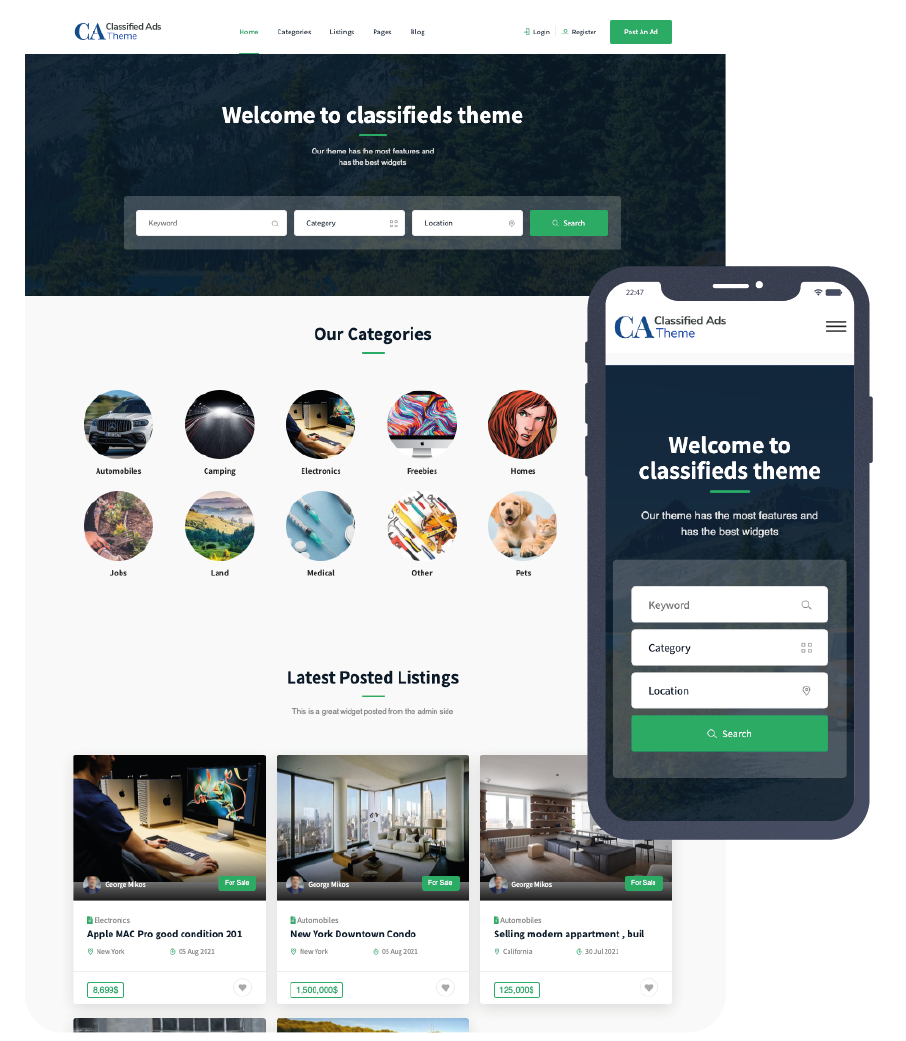The image displays an online webpage with a clean white background. At the top of the page, a prominent horizontal banner with a black background features the welcoming text "Welcome to Classifieds Team" in white. Below this banner, the phrase "Our Categories" is displayed in bold black text. Positioned underneath are two rows of five circles each, making a total of ten circles. Each circle contains a unique image, with the circle in the upper right featuring a cartoon depiction of a man with red hair. Below this section, the heading "Latest Posted Listings" is written in black text. Following this, there are three rows consisting of three images each, showcasing various indoor scenes.